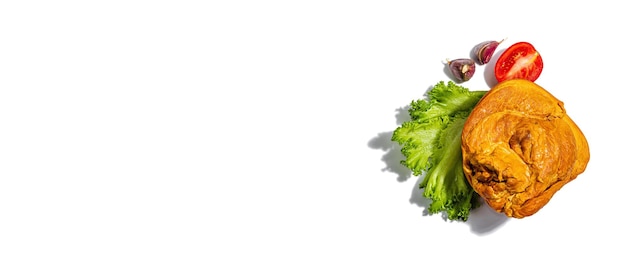This image features a top-down, overhead view of a food arrangement set against a stark white background, with gray shadows cast beneath the items. At the center lies a somewhat ambiguous, round-shaped baked item that is golden-tan and lumpy, perhaps a chocolate chip cookie, croissant, or Yorkshire pie. Beneath and surrounding this mystery baked good is a vibrant green leaf of curly lettuce. To the upper part of the composition, there are two purple garlic cloves paired with a halved Roma tomato, exposing its white core and seeds. The photorealistic style and the minimalistic setup suggest this could be menu photography, showcasing a unique, albeit puzzling, portion of a meal.